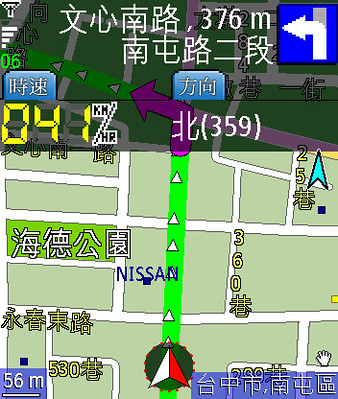The image appears to be a screenshot from a Japanese GPS or navigation system, potentially designed like a game. The interface is heavily annotated with Japanese characters and symbols, making it challenging to interpret without knowing the language. Dominating the screen is a detailed map featuring green land areas and white lines that likely represent streets. Yellow and white Asian symbols are placed alongside the streets, potentially indicating important information or landmarks. 

In the central display, directional arrows indicate navigation guidance towards north, south, east, and west. The map also displays specific distances and speed limits; for instance, there's a yellow "530" and "360," alongside associated Japanese characters, implying different metrics or points relevant to navigation. Another section shows "041 km/hr," indicating a speed of 41 kilometers per hour. 

At the top left corner, there appears to be a settings or connectivity bar. Prominently featured in blue text at the bottom is the word "NISSAN," which could suggest the user is near a Nissan facility or the system is integrated with a Nissan vehicle. Additionally, there's an icon indicating the next turn is left, reinforcing the navigational aspect of the display.